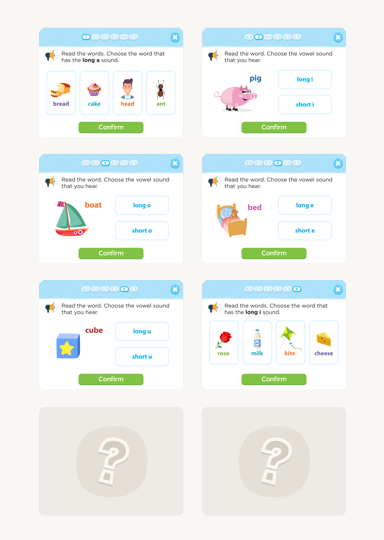This image is organized into a grid consisting of eight squares arranged in two columns and four rows. The squares in the bottom row are empty, each containing a circle and question marks. The other six squares feature a blue bar across the top and cartoon-like illustrations in the middle, with green "Confirm" buttons at the bottom.

In the top left square, there are four side-by-side illustrations labeled "bread," "cake," "head," and "ant." The adjacent square to the right contains a pig at the top and two blocks labeled "long one" and "short one."

Moving to the second row, the left square displays a sailboat labeled "boat," while the right square shows a twin-sized bed labeled "bed."

In the third row, the left square features a cube with a yellow star on it labeled "cube," and the right square contains four side-by-side illustrations of a rose, milk, a kite, and cheese, respectively.